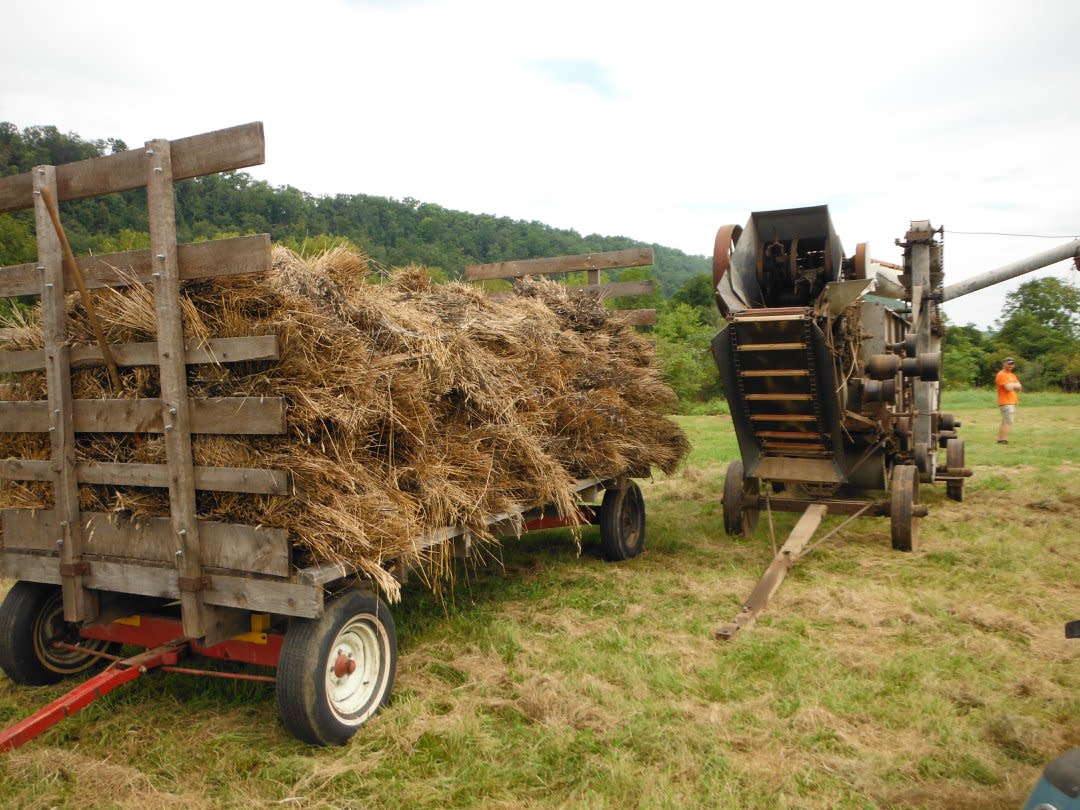This is a detailed outdoor color photograph taken during the day in a field with a mixture of green and brown grass. The scene shows a classic farm setting with various pieces of equipment and a man overseeing the area.

In the foreground on the left is a robust hay wagon. The wagon has a sturdy metal red frame and four black wheels with white rims. It has wooden slatted walls on the front and back, but the sides are open, allowing a clear view of the fresh hay piled high inside. The hay appears to have been recently cut and is a mix of golden-brown tones. 

Adjacent to the wagon, towards the right, is a piece of farm machinery, possibly a hay baler or a shredder. This machinery is also on four wheels and has several metal components, with a conveyor-like structure suggesting its function related to hay processing.

In the background to the right, a man stands with his arms crossed. He is dressed in a bright orange t-shirt, khaki shorts, dark shoes, sunglasses, and a dark baseball cap. His stance and attire suggest he may be supervising or taking a break after working with the equipment.

The backdrop features a treeline that stretches across green hills, indicating the edge of a wooded area. The sky overhead is cloudy, casting a diffuse light over the scene, typical of an overcast day. The entire setting exudes a rustic, hardworking atmosphere that is emblematic of rural farm life.